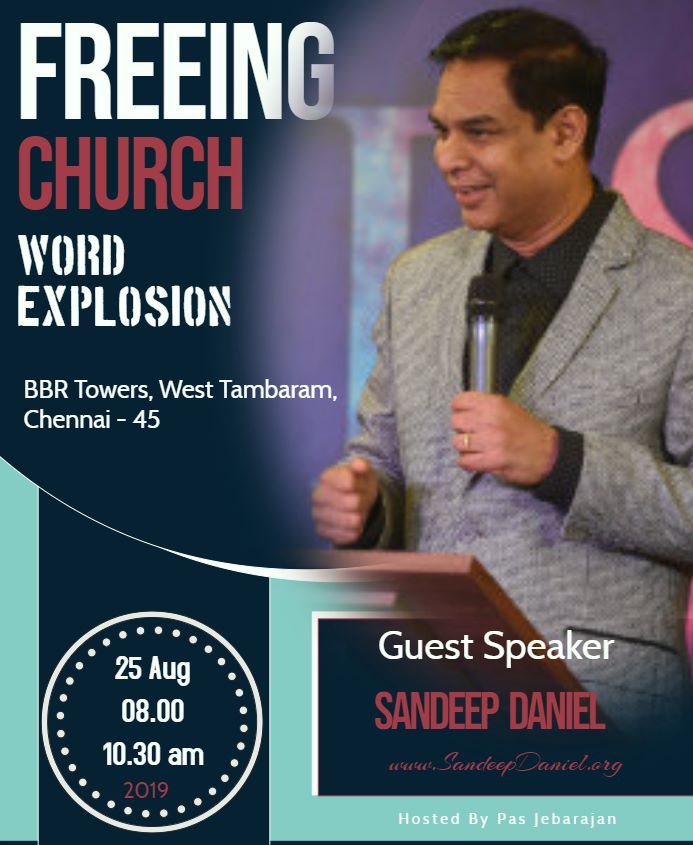Promotional Flyer for an Event at Freeing Church

The flyer is divided into two main sections. On the left, it lists important details about the venue and event. The flyer reads "Freeing Church, World Explosion, BBR Towers West, Tambaram, Chennai - 45." These details are clearly laid out against a background design that alternates between light blue and dark blue shades.

On the right, there is a picture of an Indian man with black hair, dressed in a grey suit over a black dress shirt. He is holding a microphone and appears to be speaking. The image suggests he is one of the key figures of the event.

At the bottom of the flyer, the date and time of the event are specified: "25th August, 8:00 - 10:30 AM, 2019." These details are placed in a prominent position, ensuring they catch the reader's eye.

The name of the guest speaker, "Sandeep Daniel," is highlighted in red, which stands out against the otherwise white text. His name is also accompanied by his website, "www.sandeep.org." A watermark at the bottom indicates that the event is hosted by "Paz Jebbarajan."

Further emphasizing the church's involvement, the word "church" is also printed in red, providing a striking contrast to the light and dark blue design elements that dominate the flyer. 

Overall, the flyer is visually appealing and effectively communicates all the essential information about the upcoming event.